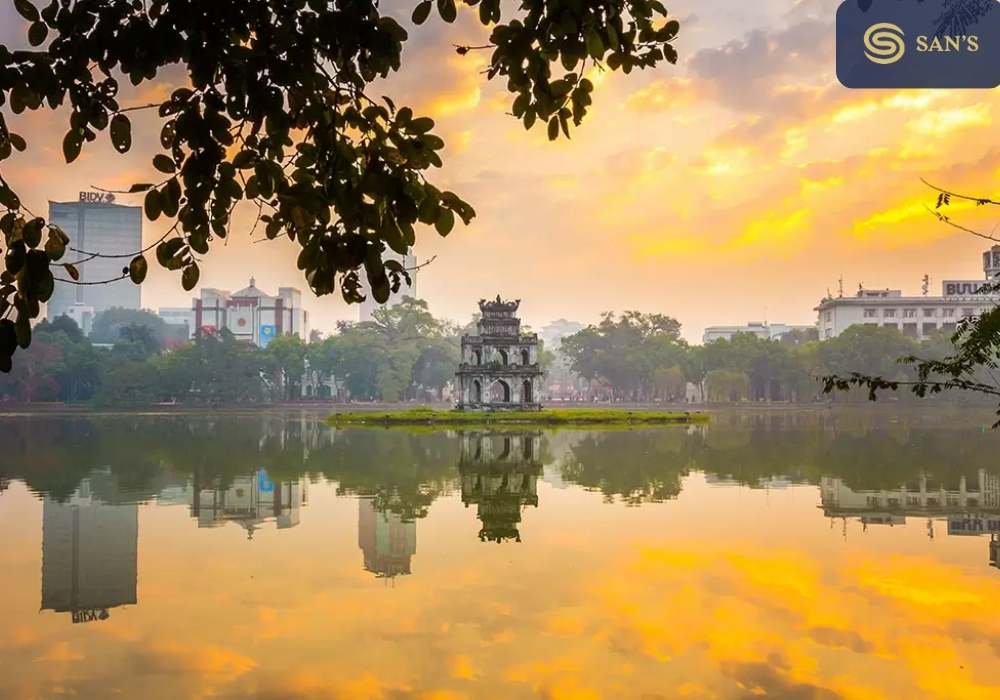The photograph captures an exotic Asian city skyline beautifully reflected in a calm lake, creating a near-perfect mirror image between the upper and lower halves. The serene water showcases a colorful sky with a setting sun and yellow clouds. A small island with a tiered pagoda-like structure stands in the middle of the lake, surrounded by greenery and shrubbery. Behind the lake, a variety of buildings, including traditional Asian architecture, modern skyscrapers, offices, and relaxation spots, dominate the skyline. On the far left, a taller building that resembles a casino is visible, along with shorter structures and a hotel-like building on the right. In the foreground, tree branches hang down, framing the scene, and the names "Sands" in a blue shaded square is noted in the top right corner. This detailed composition captures both modern and traditional elements, illustrating the peaceful coexistence of nature and architecture.